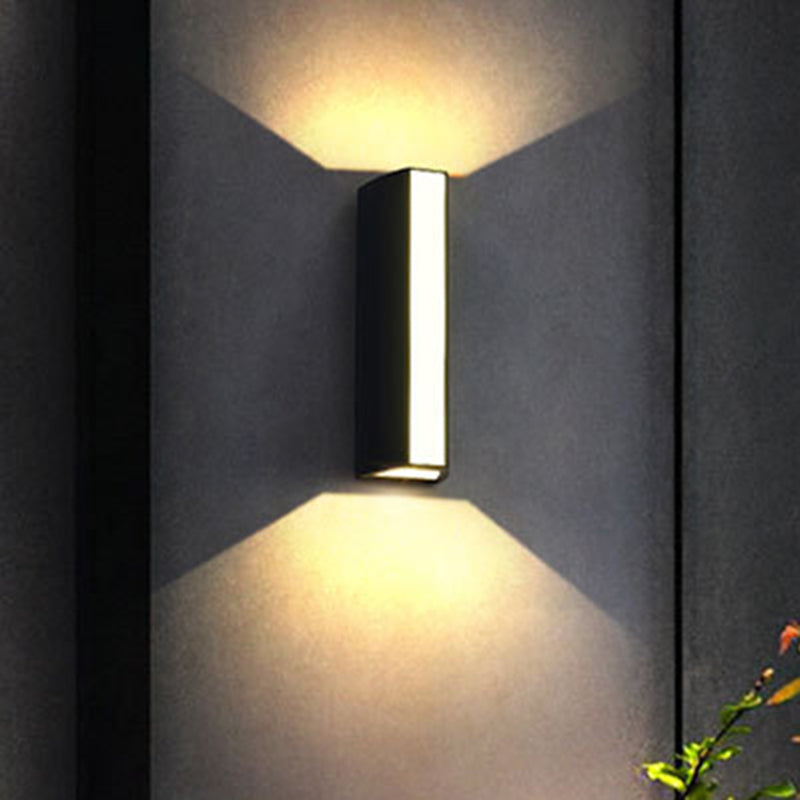The photograph features a modern, rectangular trapezoidal prism-shaped wall sconce with black sides and a white vertical center. The light it emits from the top and bottom creates striking trapezoidal beams of light on the dark grey wall, forming an intriguing visual effect resembling cat ears or a bow. The wall has a black border on the left, and a plant with green leaves and a red top is visible in the very bottom corner.